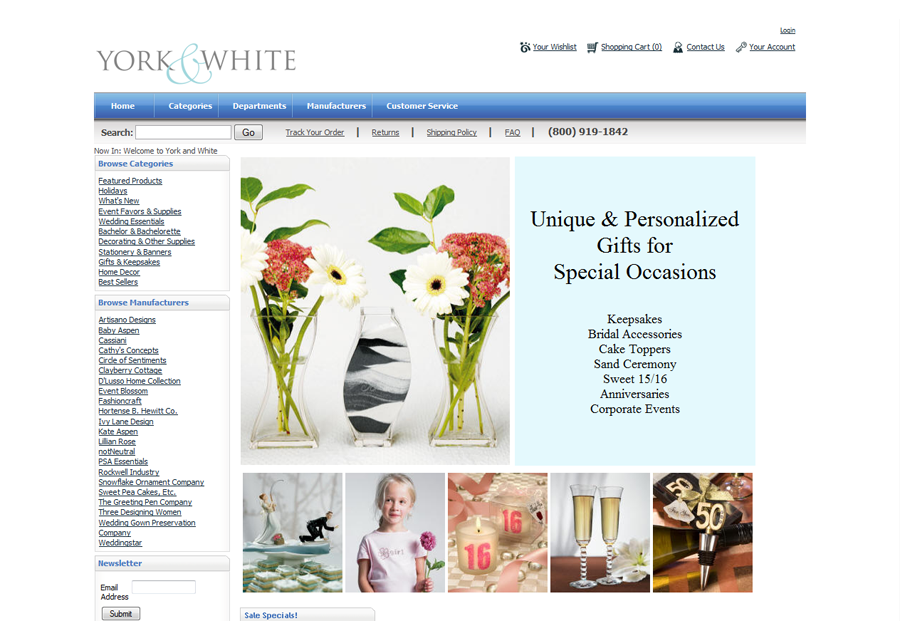This is a detailed description based on the provided voice caption:

---

**York and White Gifts Webpage Screenshot**

The screenshot captures a webpage dedicated to gifts, branded "York and White" in the top left corner. A prominent blue banner runs horizontally across the top, featuring navigation tabs for Home, Categories, Departments, Manufacturers, and Customer Service. Directly below the banner, a search bar is present but remains empty. The top section also includes links for order tracking, returns, shopping policy, FAQ, and a phone number for customer support.

On the left side of the page, a vertical column lists various categories, including Featured Products, Holidays, Stationery and Manners, Home Decor, and more. Following this column is a "Browse Manufacturers" section, highlighting brands such as Baby Aspen, Lillian Rose, and Wedding Star. Beneath this, there is a newsletter sign-up section.

The right side of the page showcases a large image of flowers and vases with the caption: "Unique and personalized gifts for special occasions, keepsakes, bridal accessories, cake toppers, sand ceremonies, Sweet 16, anniversaries, corporate events." Below this primary image, there are five smaller photos aligned horizontally from left to right. The first photo depicts a cake topper featuring a bride and groom. The second photo shows a little blonde-haired girl holding a purple flower. The middle photo displays two candles with large pink "16" numbers on their sides. The fourth photo features two glasses filled with what appears to be wine. The final photo captures items related to a 50th anniversary or birthday celebration.